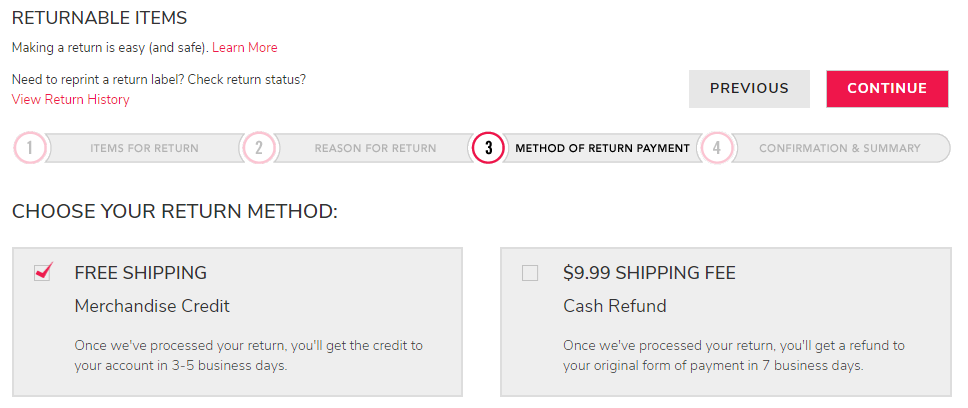This color image appears to be a screenshot from an online shopping returns page, set against a white background. In the top-left corner, there's black text titled "Returnable Items," followed by a message in smaller text that reads "Making a return is easy and safe." The words "Learn More" are highlighted in red. Below this, additional options in red text are listed: "Need to print a return label," "Check return status," and "View return history."

To the right of this section, there is a navigation box with two buttons: a grey button labeled "Previous" in black text and a red button labeled "Continue" in white text.

Directly underneath, a long grey progress bar displays four red-outlined circles with white backgrounds, each numbered 1 through 4. The first circle is labeled "Items for Return" and is greyed out, the second is "Reason for Return" and is also greyed out, the third circle, labeled "Method of Return Payment," is highlighted to indicate the current step, while the fourth circle, "Confirmation Summary," remains greyed out.

Below the progress bar, there is a heading in black text that reads "Choose Your Return Method." Two grey rectangles are positioned side by side, each containing return options with black text. The left rectangle features a red tick box for "Free Shipping" with the details, "Merchandise credit: Once we’ve processed your return, you’ll get credit to your account in three to five business days." The right rectangle outlines an alternative option with a non-ticked box, stating "£9.99 Shipping Fee." This option promises a "Cash Refund: Once we’ve processed your return, you’ll get a refund to your original form of payment in seven business days."

This detailed screenshot evidently represents the return process for an online shopping retailer, with the user currently navigating the "Method of Return Payment" step.